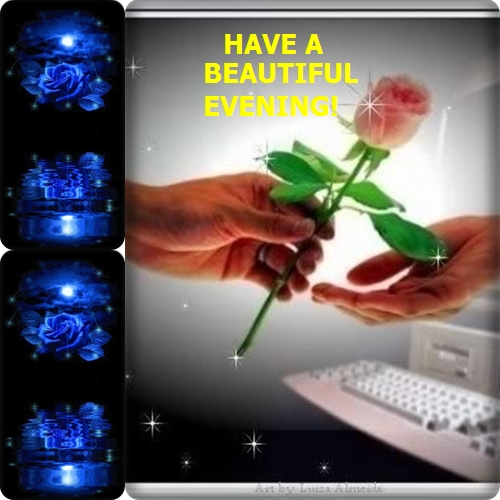The image showcases a serene nighttime scene with a background comprising two black rectangles on the left-hand side, resembling cell phone screens that display pictures of illuminated blue roses. Accompanying the roses is a dark sky backdrop featuring a white moon. On the right-hand side of the image, the words "Have a beautiful evening" are visible in centered yellow text. The image's focal point is two hands, one belonging to a man and the other to a woman. The man's hand, palm facing forward, is holding a pink rose that sparkles at its edges. The rose is angled approximately 45 degrees from lower left to upper right, as he extends it towards the woman's outstretched palm. Below the woman's hand, an old white computer keyboard and part of a computer can be seen, contributing to the setting's nostalgic feel.